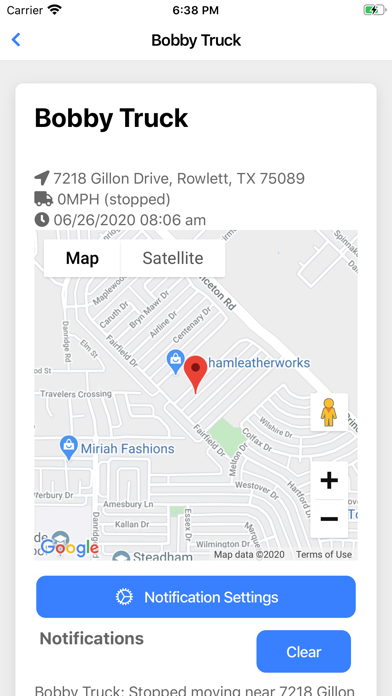A screenshot displaying a map with a white background, taken at 6:38 PM. The central focus is on a label indicating "Bobby Truck," which is currently stopped near 7218 Gilland Drive, Roulette, Texas, 75089. The label also specifies the time and date as 8:06 AM on 06/26/2020. 

The map is labeled with "Map" in bold text at the top, alongside an option for "Satellite" view and a location symbol. A blue rectangle, containing a settings icon, also appears on the screen. Within this rectangle, "Notification Settings" is displayed in black text, with the word "Clear" written in white. 

Additionally, there is a charge symbol on the battery icon, indicating the device's battery status. The information, combined with the stopped status of Bobby Truck, suggests a stationary position near the referenced address, as visually represented on the map.